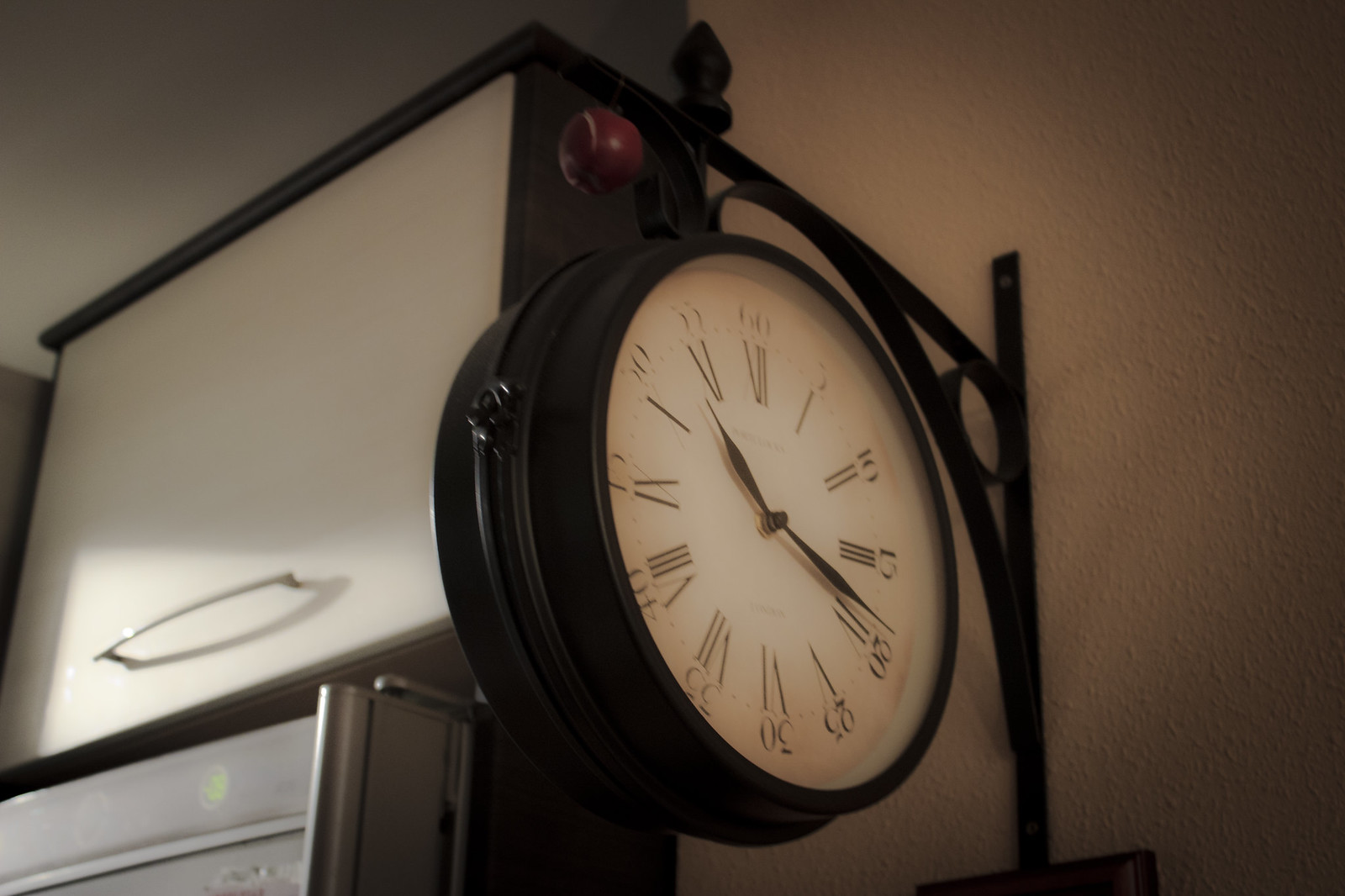This nighttime photograph showcases an old-fashioned, large, black hanging clock mounted on a perpendicular, black metal bracket attached to a rendered beige wall. The clock, reminiscent of those found in railway stations, features a white face adorned with black Roman numerals and an outer circle of minute markers ranging from 5 to 60. The numbers are black, and the clock hands are black, with the shorter hand positioned between 10 and 11 and the longer hand between 3 and 4. Behind the clock, a white cabinet with a metal handle trimmed in black is visible, adding depth to the composition.